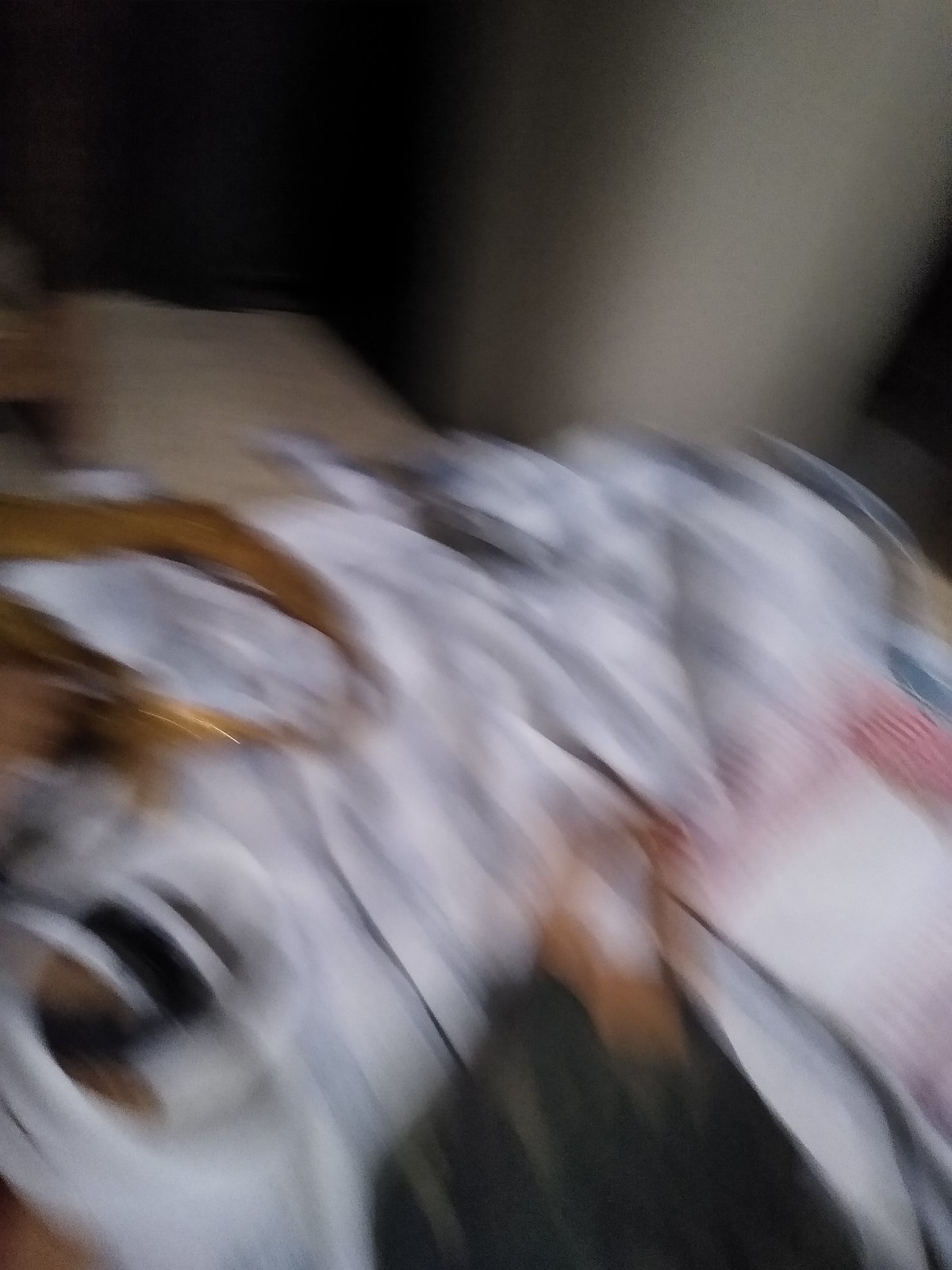The image, although blurred, captures a chaotic scene of clothes haphazardly tossed onto a surface, possibly a table or a bed. Dominating the center are white fabrics with distinct horizontal strips interspersed throughout. Among the white fabrics, a black garment, perhaps a shirt, is partially visible. In the foreground stands a large, thick gray pole, resembling those typically found in utility or furnace rooms, starkly contrasting against the entirely black background. The overall composition exudes a sense of disorder against the starkness of the dark space behind.